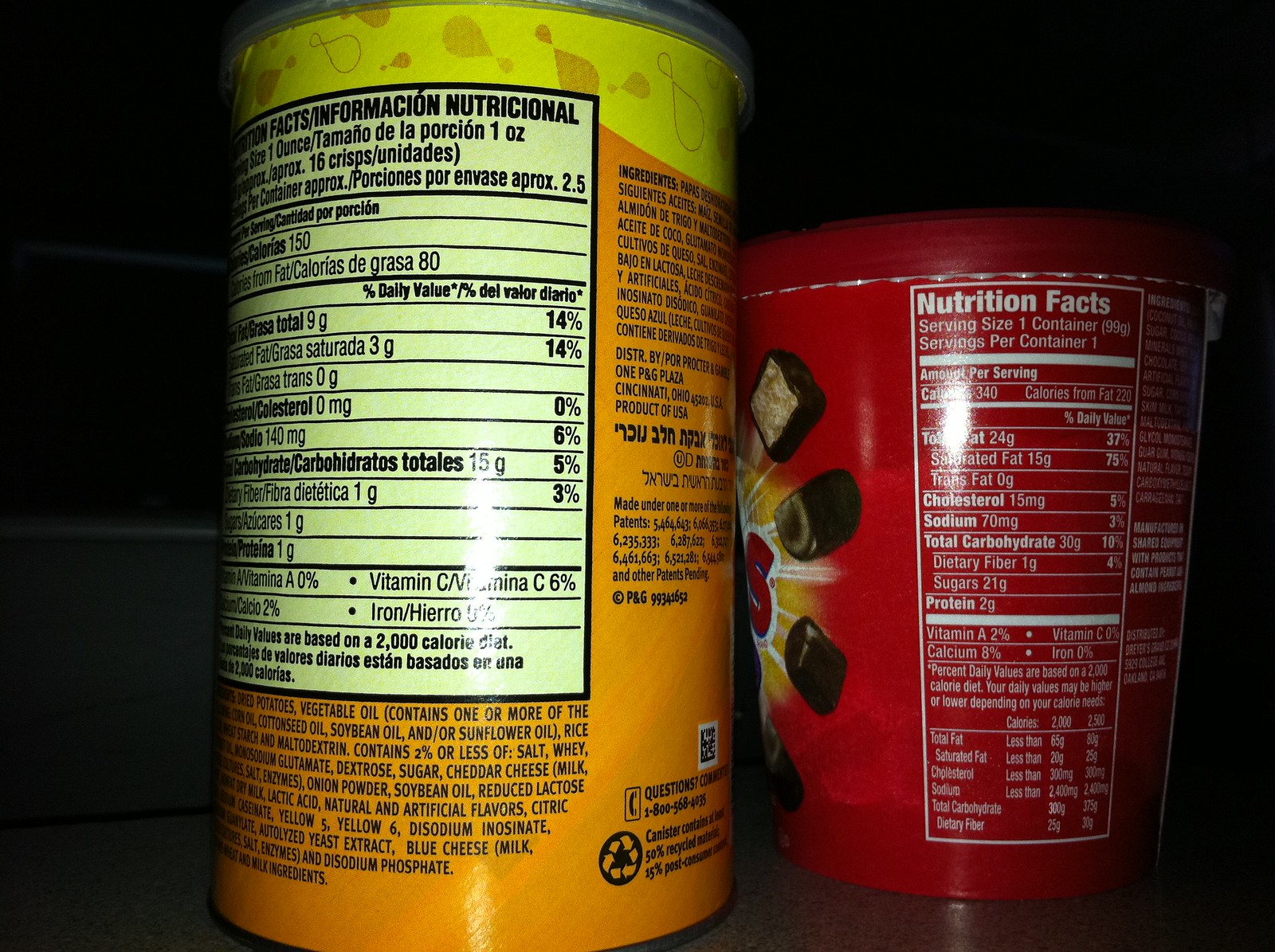In the image set against a nearly pitch-black background, we observe two distinct containers positioned on what appears to be a dark shelf. The first container, on the left, is primarily orange, transitioning to bright yellow at the top. It features a nutrition label primarily in Spanish, detailing ingredients and warnings. The second container on the right is slightly shorter, reaching about 75% of the image height, and is red with a clearly visible Nutrition Facts label in English and Spanish. This container is identifiable as Dibs ice cream due to the partial visibility of the distinctive "S" and the image of the dipped ice cream treats on the packaging. Both containers are illuminated by a flash, causing bright highlights that contrast starkly with the otherwise dark setting. The overall clarity of the text is hindered by the lighting and the mixed languages, but the general appearance suggests packaged food products, with the left possibly being a different type of snack, such as chips, given the listed ingredients and logos.